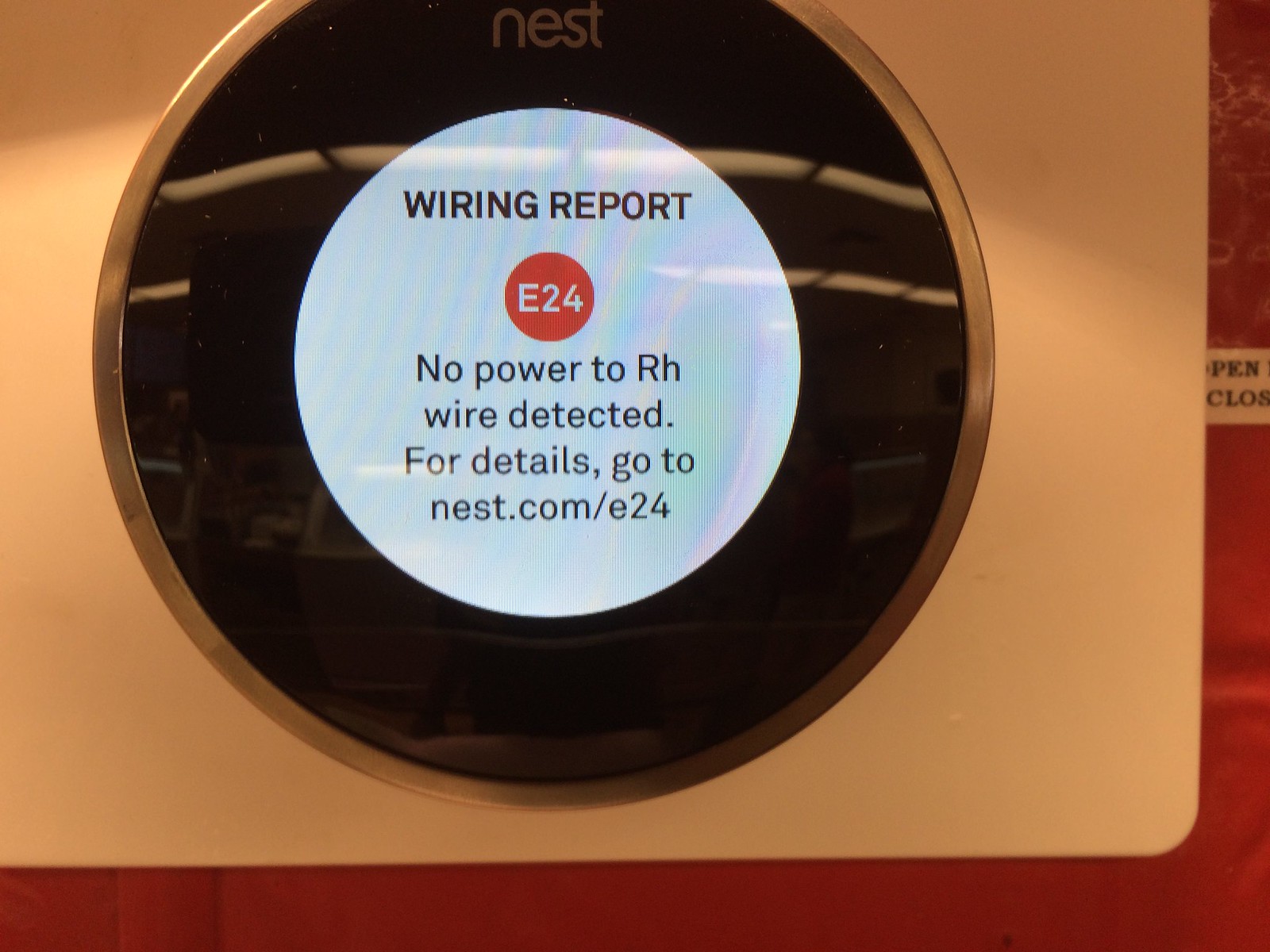The image is a close-up photograph of a digital device, specifically a Nest thermostat, mounted on a white wall. The thermostat itself is circular in shape and predominantly black. At the top of the device is the brand name "Nest" printed in a grayish-white color. Central to the thermostat is a prominent display screen that shows a warning message. The main text on the screen reads "Wiring Report" in black letters. Below this, within a smaller red circle, it shows the error code "e24." Further down, the message continues in black text: "No power to RH wire detected." For more information and troubleshooting, it directs to "nest.com/e24."